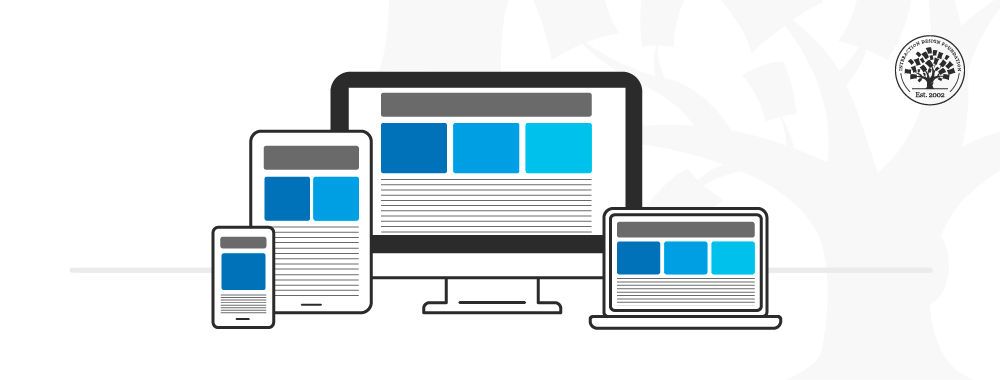This highly stylized digital illustration, reminiscent of CGI or pictograms, features several electronic devices prominently displayed against a minimalist backdrop. At the center, a desktop computer, laptop, tablet (both in horizontal and vertical orientations), and a mobile phone are all propped up to face the viewer. On each screen, a simplistic depiction of a website is rendered using colored squares and black lines to represent text, accompanied by a consistent gray bar across the top and three blue-shaded rectangles beneath.

In the upper right corner, a barely legible logo depicts a tree and includes the text "established in 2002," likely representing the company's emblem. This logo stands out in black and white, contrasting against a subtle, faint gray watermark of a different tree design that blends into the background.

The image is devoid of realistic details, focusing instead on a clean, schematic representation to emphasize the compatibility of the depicted website layout across various devices.